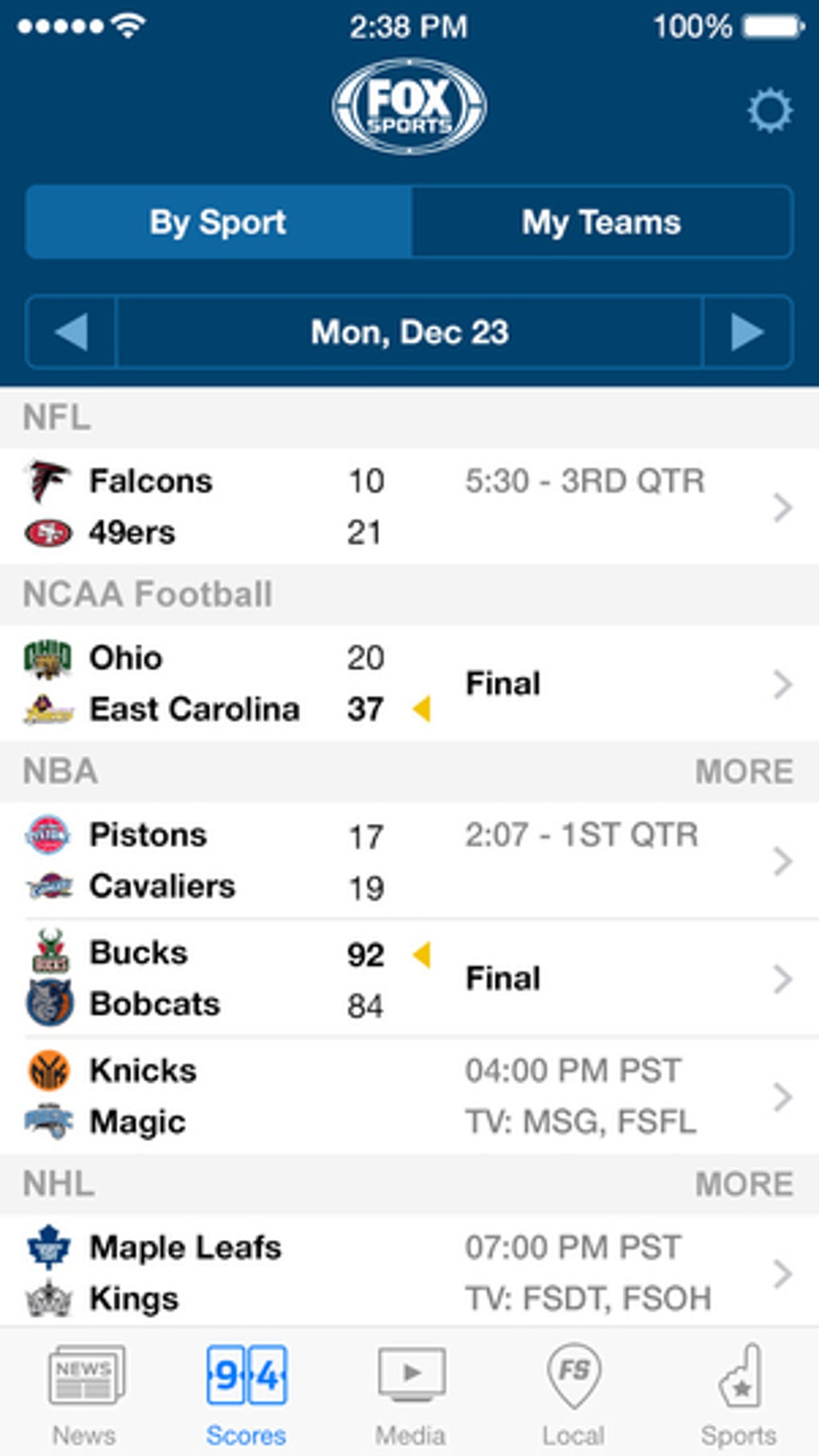The screenshot of a mobile device displays various status indicators and sports scores. At the top left corner, the network signal strength is shown with all 5 bars filled, indicating maximum signal. Next to it, the Wi-Fi signal strength is also full with 3 bars. The center of the top bar shows the time as 2:08 PM. On the top right, the battery icon indicates a full charge at 100%.

Below the status indicators, the main content displayed is related to sports, specifically from Fox Sports. It features game results dated Monday, December 23. The scores are as follows:

- Atlanta Falcons: 10 vs. San Francisco 49ers: 21
- Ohio: 20 vs. East Carolina: Finals
- Peace Team: 17 vs. Cavaliers: 19
- Milwaukee Bucks: 92 vs. Charlotte Bobcats: 84